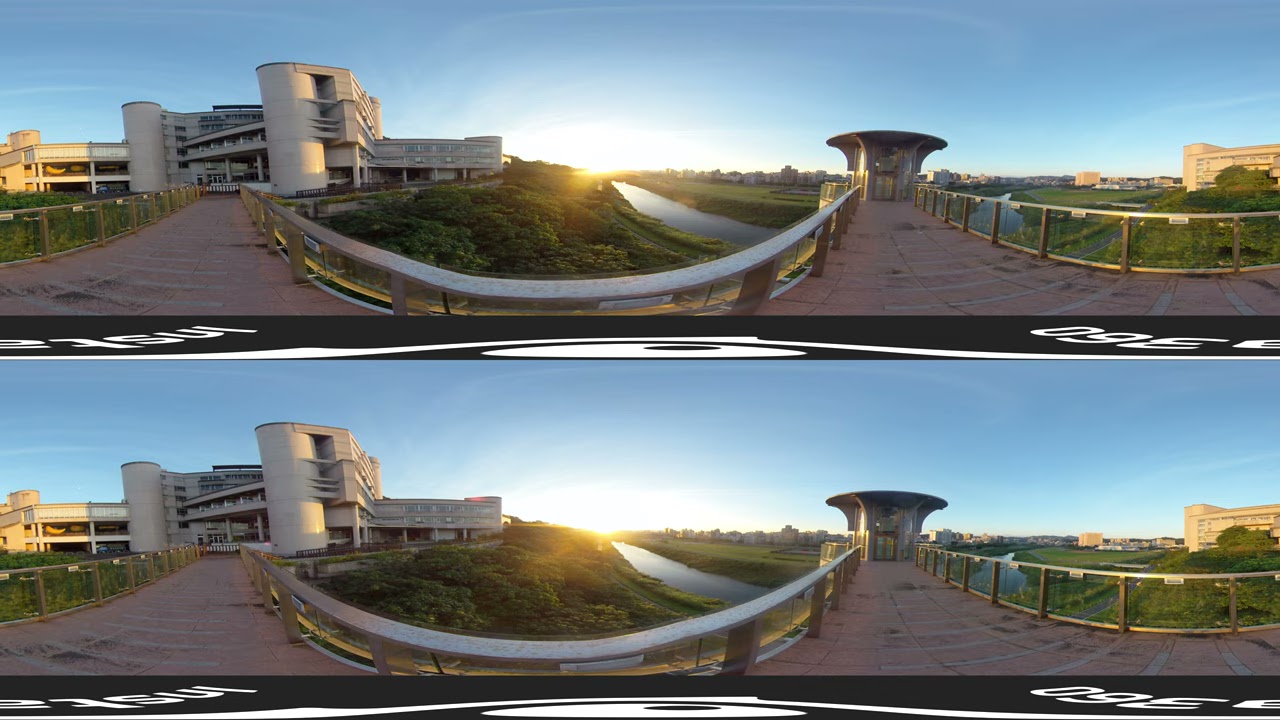The image, a color photograph in landscape orientation, features two identical panoramic views stacked one on top of the other, each with a fisheye effect. Dominating the left side of the photo is a large modern commercial building with white exterior walls and two prominent cylindrical structures, possibly spiral staircases, which resemble parking garages. This building is accompanied by a wood plank path and green landscaped area on a gentle slope.

In the center, the photograph captures a serene river flowing from the right side into the distant horizon, where the sun, appearing white, is either rising or setting against a clear blue sky. Green bushes and grass border the waterway, adding a lush, natural feel to the scene.

To the right, the image displays another structure with a circular roof at the end of a wood plank walkway, encircled by gray railings and black beams. Adjacent to this is a beige stucco building. In the background, more buildings and additional streams of water with green vegetation can be seen, although they are partially obscured.

The ground in the photographs appears reddish or light gray, and below each panoramic view are technical details presented in white text on a black background, including the number "360". The overall scene is outdoors and could depict an institutional setting, possibly resembling a school or hospital, with a picturesque and detailed representational realism enhanced by panoramic filters.